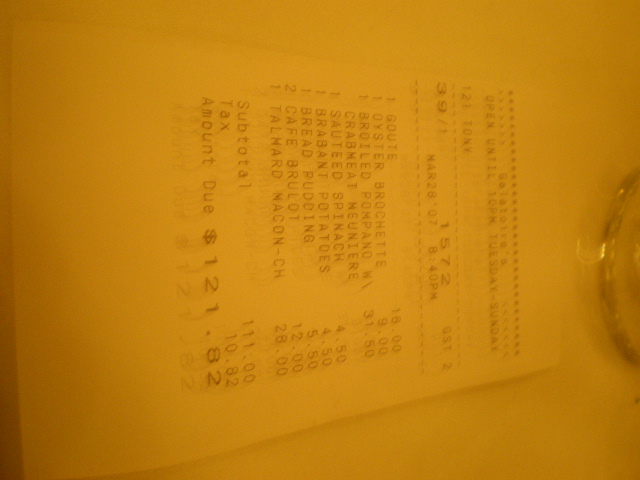The image displays a receipt from a place named Galatoriatà, which is open from Tuesday to Sunday until 10 PM. The receipt is angled diagonally with the top part positioned to the right and the bottom to the left. The image features a bright yellow filter that casts a yellowish tint over the entire scene, including a goldish half-circle, possibly a bracelet, visible at the top right. The receipt itself blends into the background, making it challenging to read. At the top, following a series of asterisks, vendor information is printed. The timestamp shows March 26, 2007, at 8:40 PM. Barry ordered 9 items, totaling $111.00, with an additional tax of $10.82, bringing the total amount due to $121.82. The list of items includes sautéed spinach and other dishes written in a language that might be French.